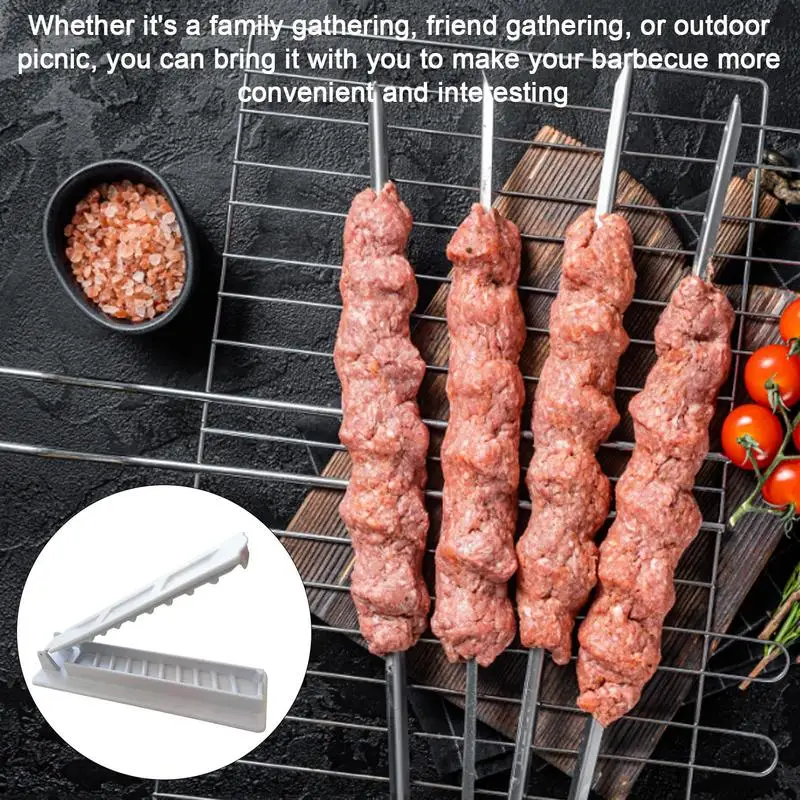A top-down photograph showcases a barbecue setup featuring a grill rack resting on a dark brown wooden chopping board. On the rack, four thick, metal skewers are laden with raw, minced meat, potentially beef. To the right of the grill rack lies a vibrant vine of five small, bright red cherry tomatoes. On the left side of the image, there's a small black bowl filled with Himalayan pink salt. The entire arrangement sits atop a rough-textured, black stone or stucco surface. In the bottom left corner, a white circular kitchen device, possibly a meat tenderizer, is visible with its lid open, showing raised horizontal lines inside. The background includes a white text in a plain font that reads: "Whether it's a family gathering, friend gathering, or outdoor picnic, you can bring it with you to make your barbecue more convenient and interesting." This appears to be an ad for a portable skewer grilling kit.